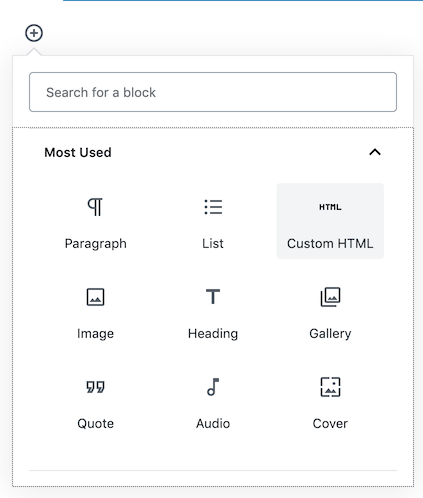This image depicts a screenshot of a small interface window, likely from a computer or cell phone. The window features an all-white background. In the top left corner of the window, there's a circular button with a plus symbol in the center, indicating it can be pressed. Directly below this button is a search bar with the placeholder text "Search for a block."

Below the search bar lies a square-shaped section labeled "Most Used." This section contains a 3x3 grid of nine buttons, each representing different functions. 

- The top row from left to right includes: a "Paragraph" button, a "List" button, and a "Custom HTML" button.
- The middle row features: an "Image" button, a "Heading" button, and a "Gallery" button.
- The bottom row comprises: a "Quote" button, an "Audio" button, and a "Cover" button.

Each button is designed for quick access to commonly used features in the software or application.